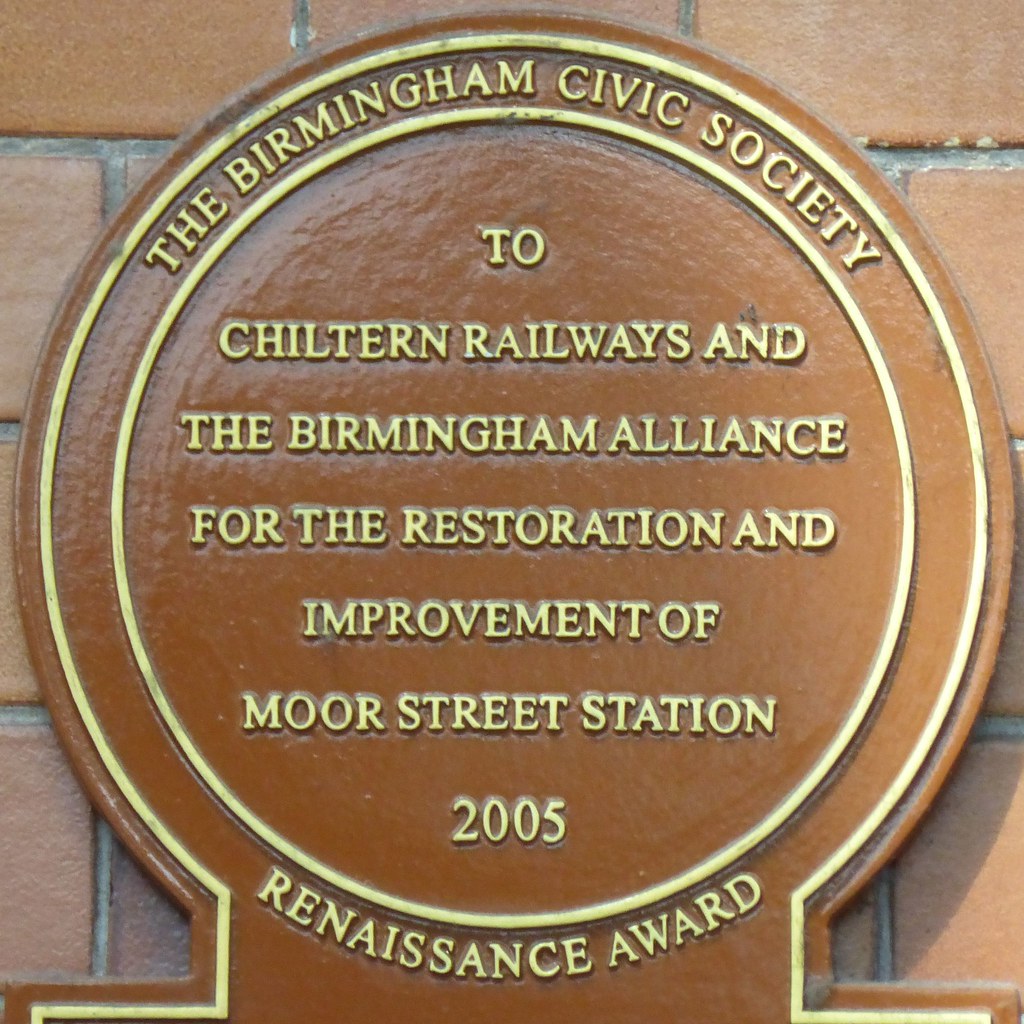The image depicts a round, brown plaque affixed to a rust-colored brick wall, likely outside as sunlight illuminates the sign. The plaque, which appears to be made of metal, is outlined with a yellow circular line and is inscribed with gold text. At the top, it reads "The Birmingham Civic Society" in a curved format. Below, in the center, it states, "Two Chiltern Railways and the Birmingham Alliance for the Restoration and Improvement of Moore Street Station, 2005." At the bottom, outside the central circle, the text "Renaissance Award" can be read. The overall effect suggests the plaque commemorates an award for a joint restoration and improvement project of Moore Street Station. The image is significantly zoomed in, cutting off the lower portion of the plaque, thereby limiting the view to only the described details.